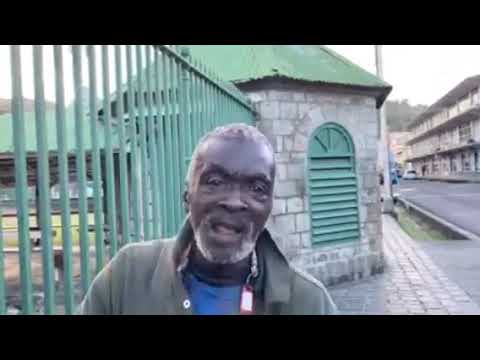This is a color photograph framed with black widescreen bars at the top and bottom, depicting an older, dark-skinned African-American man who appears to be in mid-speech, looking at the camera. He has short, gray hair and a matching gray beard and mustache. The man is dressed in a green, button-up jacket over a blue shirt with a black collar. Directly behind him is a green metal fence with vertical slats, which extends above his head. Attached to the fence is a stone building with green, arched window shutters and a pointed, green metal roof. This building has a hexagonal shape and is built from concrete or stone blocks. Further behind him, cobblestones are visible, as well as a hill with trees. To the right of the man, there is a sidewalk, a curb, and a street. A three-story building, possibly an apartment complex or shop, is seen on the right-hand side of the image against the backdrop of a white sky.